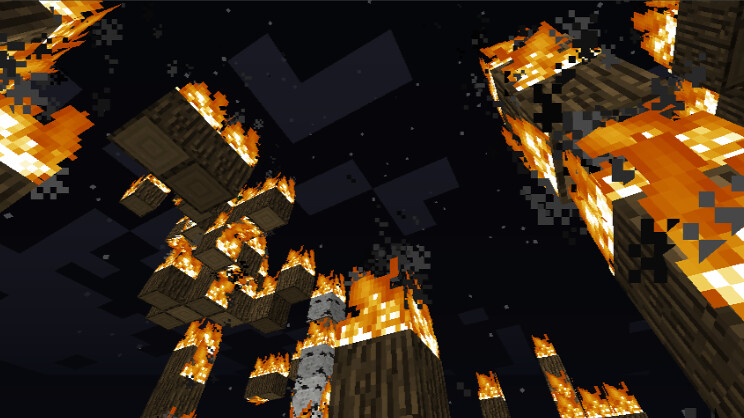This image, reminiscent of a three-dimensional video game similar to Minecraft, features a detailed nightscape constructed from a variety of cubic blocks and objects replicating physical elements from the real world. Prominent in the scene are several brown wooden pillars or towers, intricately designed with vertical lines running along their surfaces. Atop these wooden structures, square-like flames flicker with a gradient of yellow at their base transitioning to orange at their peaks, adding a dynamic and vibrant element to the image. The backdrop portrays a night sky, enveloped in darkness and dotted with various square shapes of gray, likely representing clouds. Scattered throughout the sky are numerous tiny dots, evocative of stars, lending a touch of celestial beauty to the overall scene.